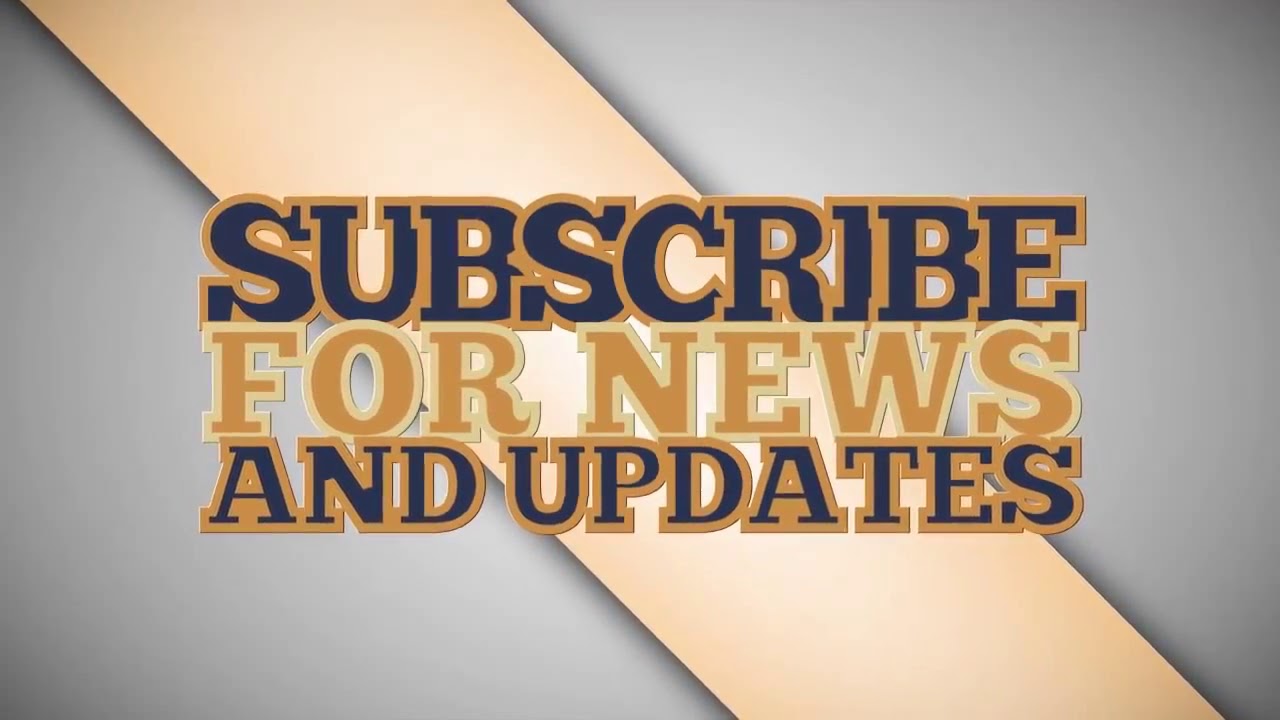The image features a medium gray background with a champagne-colored diagonal stripe running from the top left to the bottom right. In the foreground, there are three lines of text, all center-aligned both horizontally and vertically, occupying approximately 50-60% of the image's height. The first line reads "SUBSCRIBE" in dark navy blue capital letters with a golden outline. The middle line, slightly smaller, says "FOR NEWS" in a butterscotch orange color, also bordered by a light golden outline. The bottom line reads "AND UPDATES," matching the dark navy blue and gold outline of the first line. The text encourages viewers to subscribe for news and updates, reminiscent of a call to action often seen at the end of YouTube videos. Triangular patches of gray occupy the upper right and bottom left corners, completing the design.